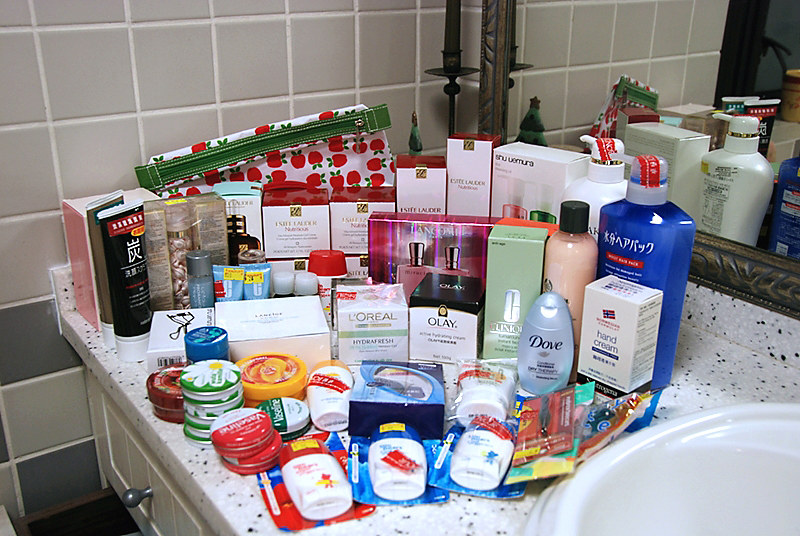In this image, the scene unfolds within a well-used bathroom. The granite countertop is inundated with an array of personal care items. The left side of the counter is cluttered with a variety of hand creams, lotions, body balms, and skincare products, organized haphazardly in boxes, tins, and containers. Renowned brands such as Dove, L'Oreal, Olay, Shu Uemura, and Estee Lauder are part of this collection, along with several items featuring Asian packaging adorned with distinct Asian characters. 

The off-white granite countertop contrasts slightly with the surrounding elements and stretches beneath a large mirror, which reflects the chaotic assortment of products. The mirror itself is framed in a dark brown, reminiscent of a classical picture frame. The bathroom walls are adorned with light gray tiles, subtly broken up by patches of darker gray tiles towards the lower left side of the image. This creates a subdued, yet elegant backdrop for the bustling countertop scene.